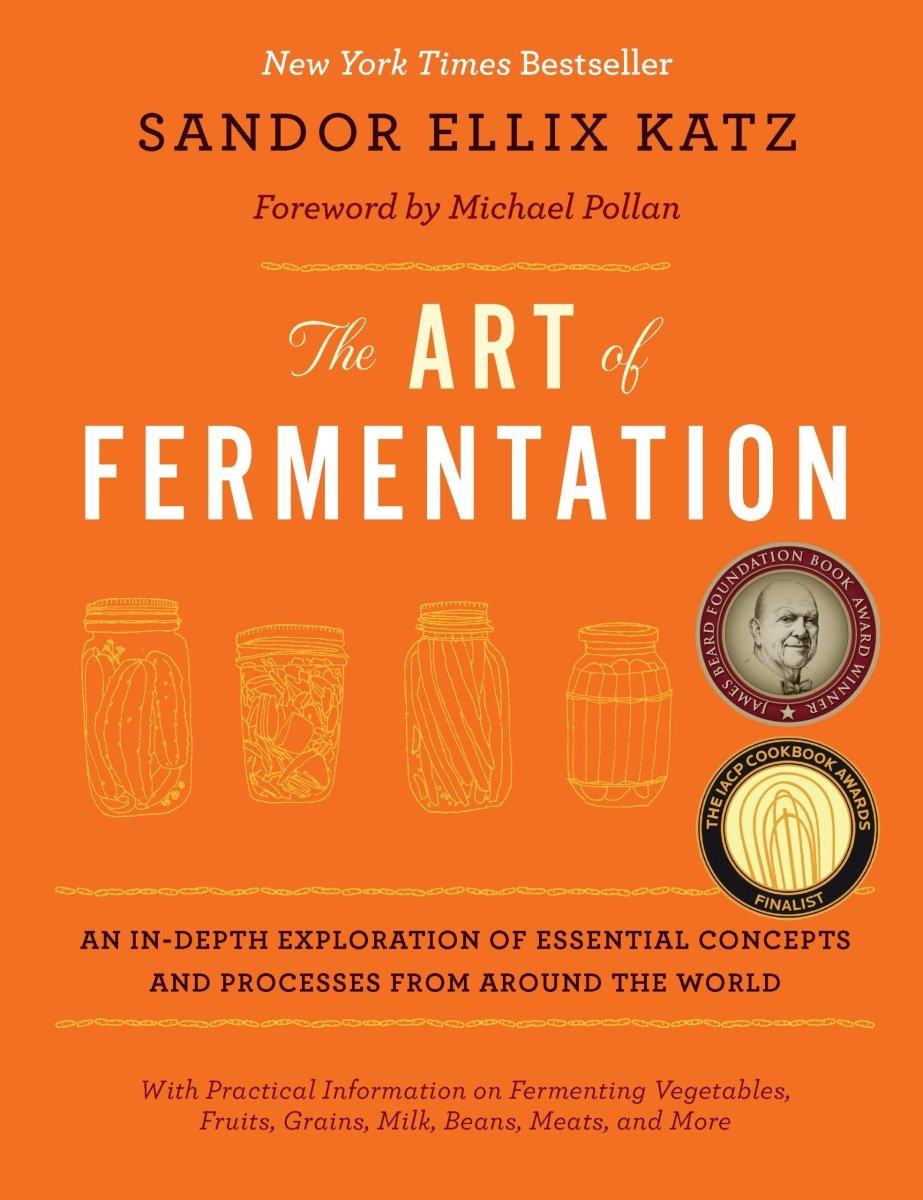This vibrant book cover, set against an orange background, highlights the New York Times Bestseller "The Art of Fermentation" by Sandor Ellix Katz. The cover features white text announcing its bestseller status, with the author's name in black and a forward by Michael Pollan in red italics. The title, "The Art of Fermentation," is prominently displayed in white text. 

Centrally placed are four yellow-outlined illustrations of canning jars, indicating the contents inside, which include cucumbers among other foods. To the right of these jars, two circular badges are displayed: the top one framed with a dark purple band, showcasing a black-and-white portrait of a smiling man and the accolade "James Beard Foundation Book Award Winner" around the edge. Below that, a similar circle with a cream interior and gold illustrations announces the book as a finalist for the IACP Cookbook Awards.

At the bottom of the cover, in black text, is a description of the book as "an in-depth exploration of essential concepts and processes from around the world." Below that, in red text, it offers "practical information on fermenting vegetables, fruits, grains, milk, beans, meats, and more." The cover skilfully combines color illustration with graphic design, effectively conveying the book's rich content and its prestigious recognitions.